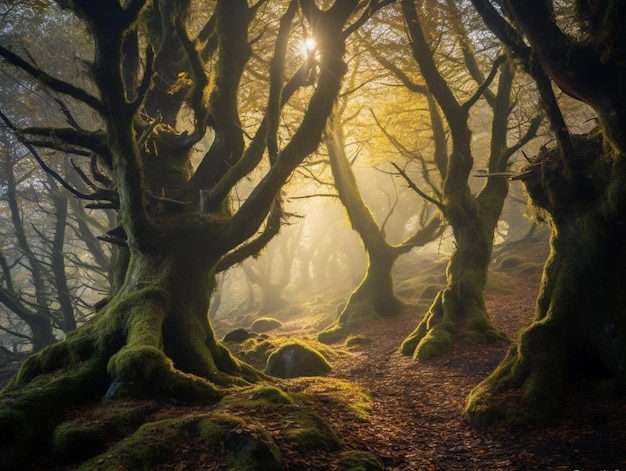The image is an enchanting painting of a foggy forest bathed in early morning light. The forest floor is a mosaic of brown leaves and small, moss-covered rocks. Central to the composition is a vast expanse of trees, with one particularly large tree trunk dominating the upper left corner. This tree is covered in green moss and boasts unusually shaped branches that extend in various directions. In contrast, three smaller trees, also moss-covered, stand to the right of the large tree, sharing similar oddly shaped trunks and limbs. The distant trees are slightly obscured by a mystical mist, adding to the ethereal quality of the scene. Sunlight filters through the canopy, creating a bright, yellowish glow that permeates the fog and illuminates the dense woodland. The entire ambiance of the painting is serene, with the interplay of light and shadow enhancing its mystical and tranquil essence.